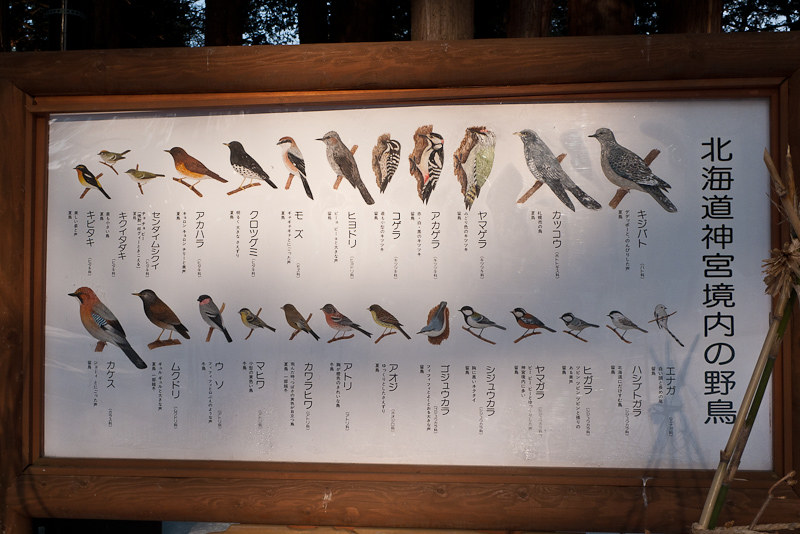This photograph captures a detailed, framed poster depicting various species of birds, positioned outdoors against a scenic backdrop of tree trunks, leaves, and a blue sky. The poster is housed in a medium brown wooden frame with a protective glass front and is oriented horizontally. Across a white background are color illustrations of birds, arranged in two horizontal rows—12 birds on the top row and 13 on the bottom, totaling 25 birds. Each bird is depicted in profile, mostly perched on branches or tree trunks, showcasing their distinct sizes, beak shapes, and plumage colors, including shades of gray, black, white, and splashes of red, orange, and yellow. Accompanying every bird illustration are vertically oriented descriptions written in Asian characters, presumably Chinese or Japanese, providing their identification and details. Prominently, large oriental characters appear on the right side of the poster. The presence of a bamboo stick with a brush leaning against the right of the frame suggests an artistic or educational purpose, possibly indicating that the poster serves as an informational guide for bird watchers or visitors at a nature preserve or park in an Asian country.